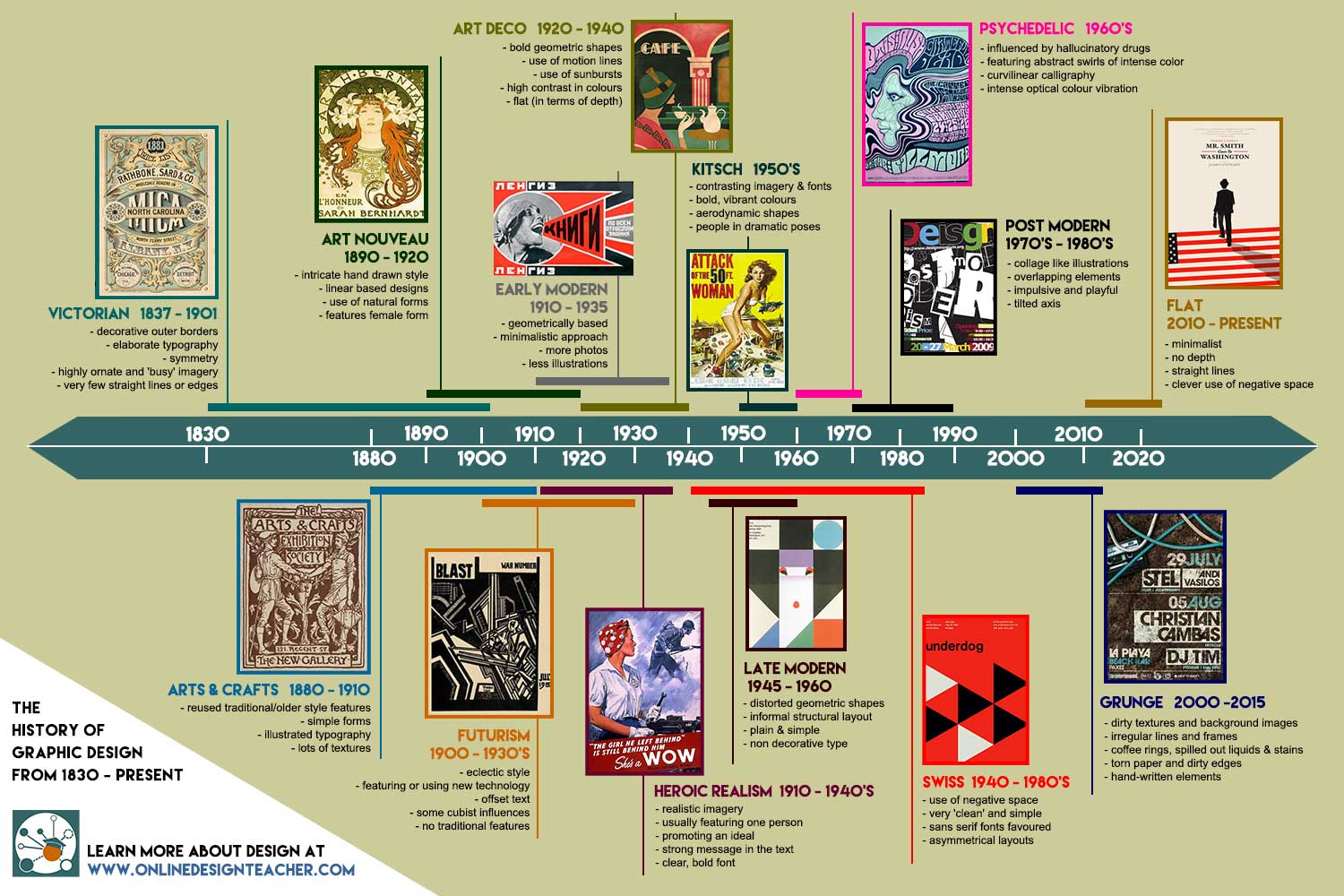The image is a detailed timeline showcasing the history of graphic design from 1820 to the present. The timeline is presented on two long green rectangles converging to a point and annotated with years from 1820 to 2020. Various images representing different design periods are aligned above and below these rectangles, correlating with their respective eras. Key design movements highlighted include the Victorian era (1837-1901), Arts and Crafts, Art Nouveau (1890-1920), Futurism, Early Modern (1910-1935), Art Deco (1920-1940), Heroic Realism, Kitsch (1950s), Late Modern, Psychedelic (1960s), Swiss (1940s), Postmodern (1970s-1980s), Grunge (2000-2015), and Flat design (2010-present). In the lower left corner, there's a white section with black text stating "The History of Graphic Design from 1820 to the Present," followed by "Learn more about design at www.onlinedesignteacher.com," accompanied by a flower logo.